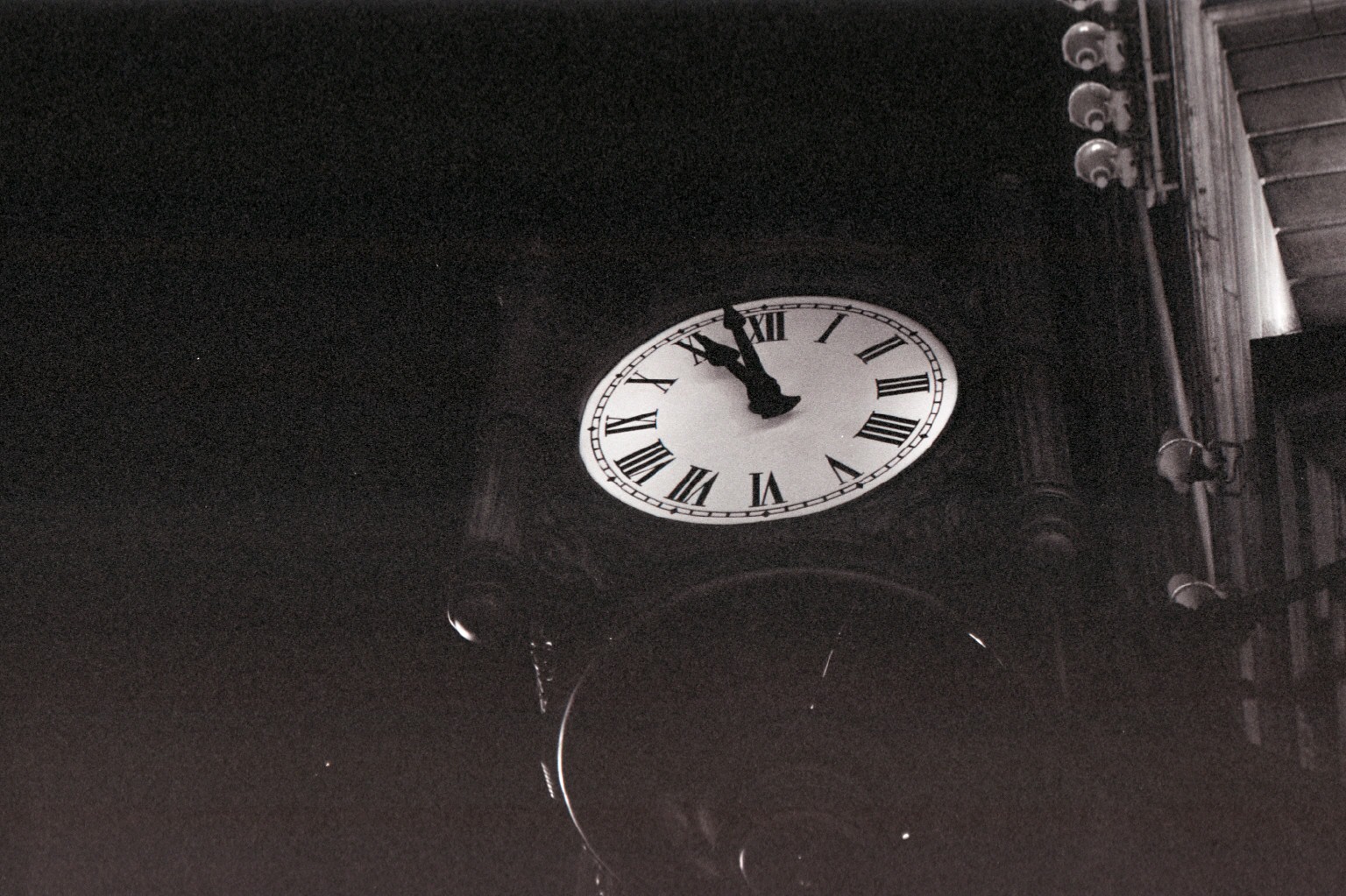This is a black and white, grainy photograph that appears to be taken at night, showcasing a clock face as its central subject. The clock, adorned with Roman numerals and set at almost 11 o'clock, is set against a stark, dark background that transitions from deep black at the top to a brownish-gray towards the bottom. Positioned in what resembles the middle of the image, the clock face itself sits within a square frame and is partially encircled by a gradient ring that fades from white to gray. 

Flanking the clock are two pillars, adding to the architectural ambiance. To the right of the clock, there is a complex, steampunk-like structure with interleaved gray components that could be interpreted as a radiator, Tesla coil, or some other mechanical element. Additional building-like features, possibly part of a street light post or metal siding, are subtly visible but hard to define due to the image's overall darkness. In the upper right-hand corner, you'll notice what appear to be white and gray keys, adding to the enigmatic feel of the composition.